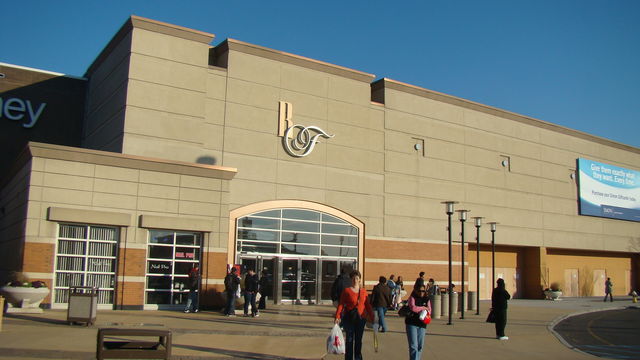The image captures a lively scene in front of a partially visible storefront reminiscent of JCPenney, characterized by its white letters with black borders. Only the letters "E" and "Y" are prominently visible, although the store's complete identity remains unclear. The main focus shifts to an adjacent storefront displaying indistinct letters which may include "B," "R," or "F," suggesting it is a lesser-known or different store. 

The building's facade features a cement-colored surface at the top, with horizontal bands of a similar hue descending towards the bottom. These bands are interspersed with sections resembling individual bricks. Near the base, the structure transitions to a darker black color, except around the window frames. The entrance of the store is clearly visible, accompanied by a light post. The bustling sidewalk is populated with numerous pedestrians, some carrying shopping bags, contributing to the overall vibrancy of the scene.